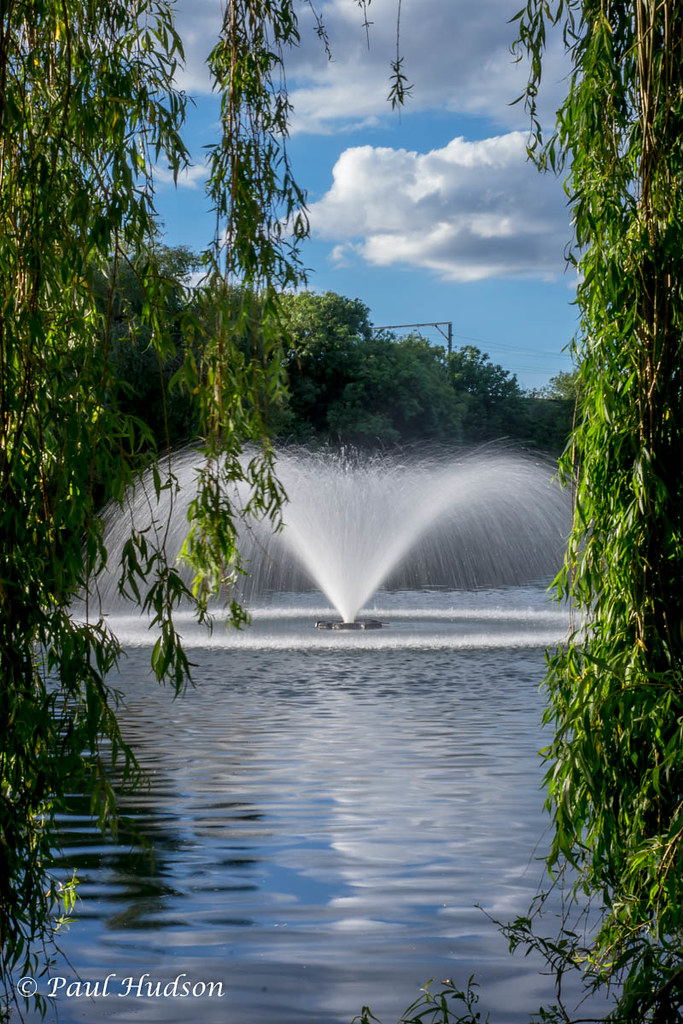This vertically aligned photograph captures a stunning fountain situated in the middle of a serene, blue pond. The water, appearing a calming mix of deep blue and white, ripples gently from the disturbance created by the fountain's strong, circular spray. Surrounding the pond, tall trees frame the scene with their lush green leaves hanging down like delicate curtains on both the left and right sides of the image. In the background, more trees add depth and greenery to the landscape. Above, the sky is a vibrant blue adorned with large, puffy white and gray clouds, casting subtle reflections on the pond’s glassy surface. In the bottom left corner, a white text with a copyright symbol reads “Paul Hudson.”